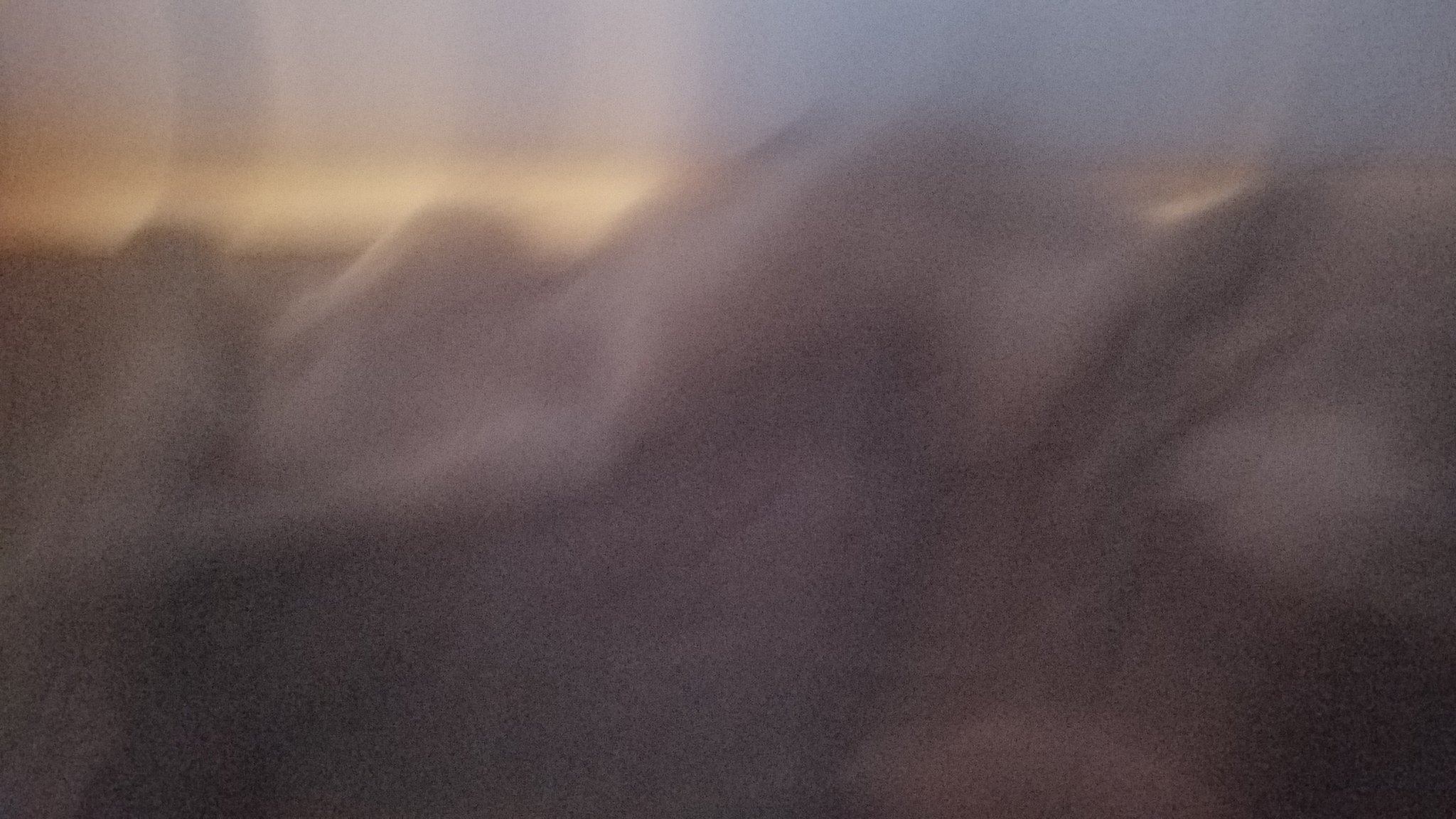This horizontally-oriented color photograph is notably out-of-focus and blurred, making it challenging to distinguish the exact subject. Dominating the bottom two-thirds of the image is a convoluted, bumpy area that might be reminiscent of a rocky landscape or folded material, vaguely shaped like mountains. This foreground area is a soft pastel purplish-beige or brownish-gray color, with light highlights that could be reflections, possibly from the sun, or due to the photograph being taken through glass. 

Above this rugged foreground, a distinct horizon line separates the lower part of the image from the soft pastel yellowish-gold strip, which might suggest a horizon or clouds lit by a setting sun. The uppermost portion of the image is filled with a very soft bluish-gray or blue color, possibly representing the sky at twilight. Despite the blur, the color gradient from blue at the top, through yellow, to the purplish-beige foreground offers an artistic and soothing effect, reminiscent of a serene landscape at sunset. The entire composition is rendered with a mysterious and abstract quality due to the extreme blurriness and apparent reflections.